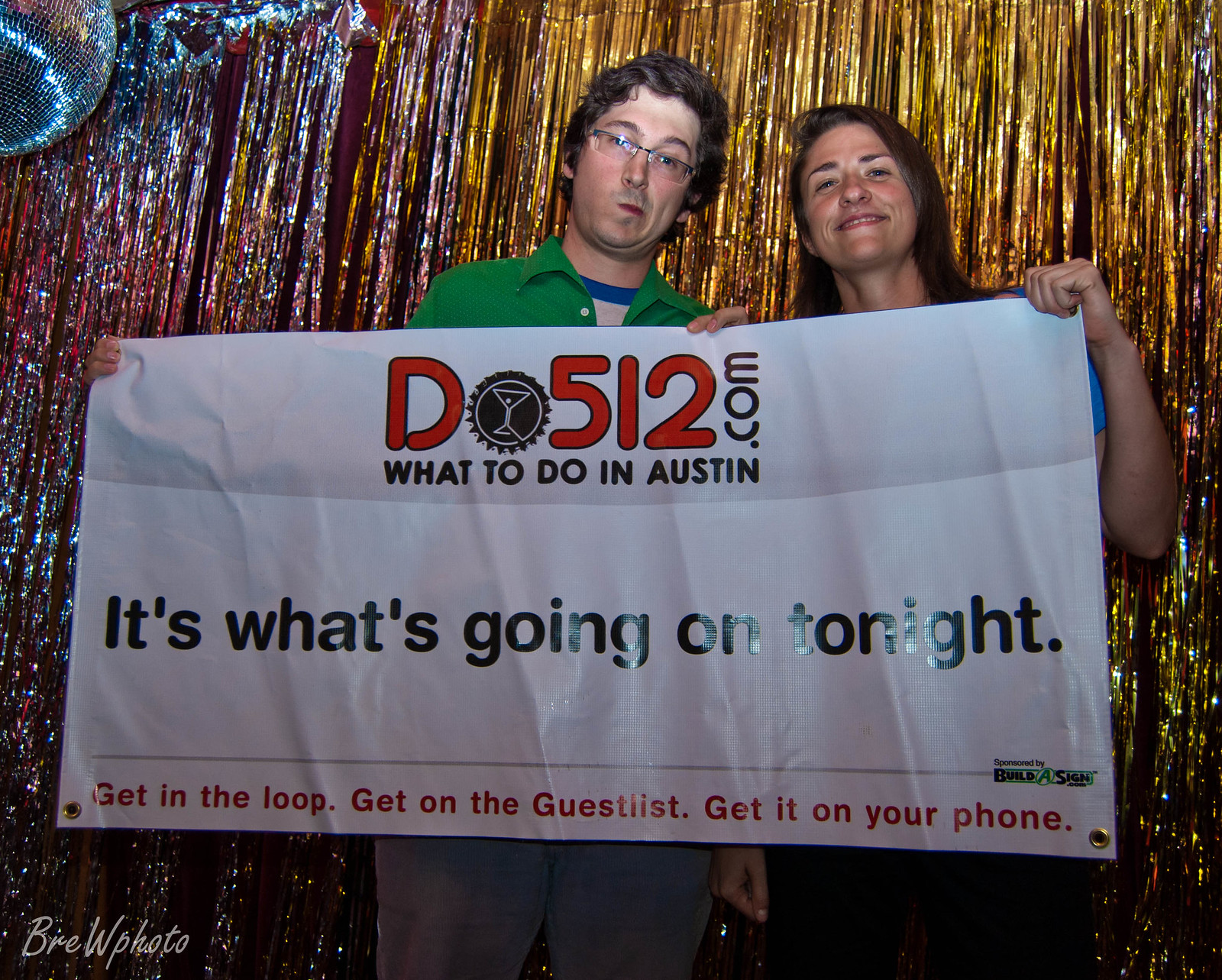The image features a cheerful young man and woman standing in front of a festive tinsel backdrop of gold and silver, with a disco ball partially visible in the upper left corner. The man, who has dark brown hair and glasses, is dressed in a green collared shirt layered over a white and blue shirt, and gray pants. The woman beside him has long brown hair and appears to be wearing a blue t-shirt and black pants, although her shirt is mostly obscured by the large white banner they are holding. The banner prominently displays the website "Do512.com" in bold red letters, with a beer cap and a martini glass integrated into the "O". Below, in black text, it reads "What to do in Austin." Centrally, it states, "It's what's going on tonight," and at the bottom in red text, it urges, "Get in the loop, get on the guest list, get it on your phone." The bottom left corner bears the mark "breed W photo" in white.